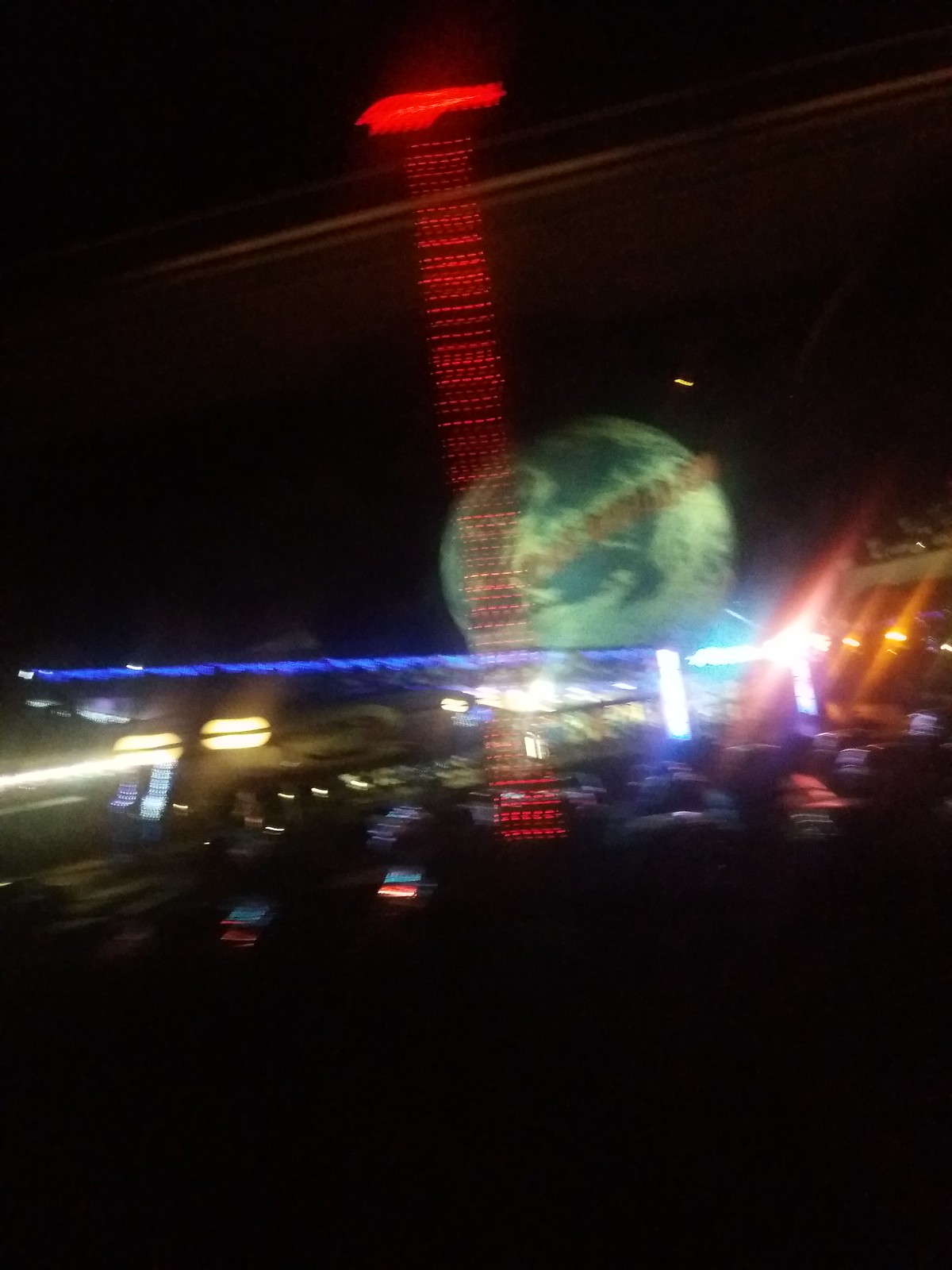Captured in the depth of night, this photograph vividly portrays a bustling parking lot in front of a dynamic venue. Dominating the background, right at the center of the frame, is the venue itself, illuminated by a striking red light that casts an ethereal glow over a spherical object depicting the Earth in blue and gray tones. Although the red lettering on this globe remains indecipherable due to the distance, it adds a layer of intrigue to the scene. Complementing this celestial centerpiece, streaks of blue and red lights zigzag across the sky, perhaps reflections or lights enhancing the atmosphere. Below, the scene is grounded by the familiar sight of car taillights, indicating cars maneuvering in and out of the parking lot. The asphalt is dotted with various vehicles, predominantly in shades of black, silver, and gray, adding to the lively yet orderly chaos of the night.